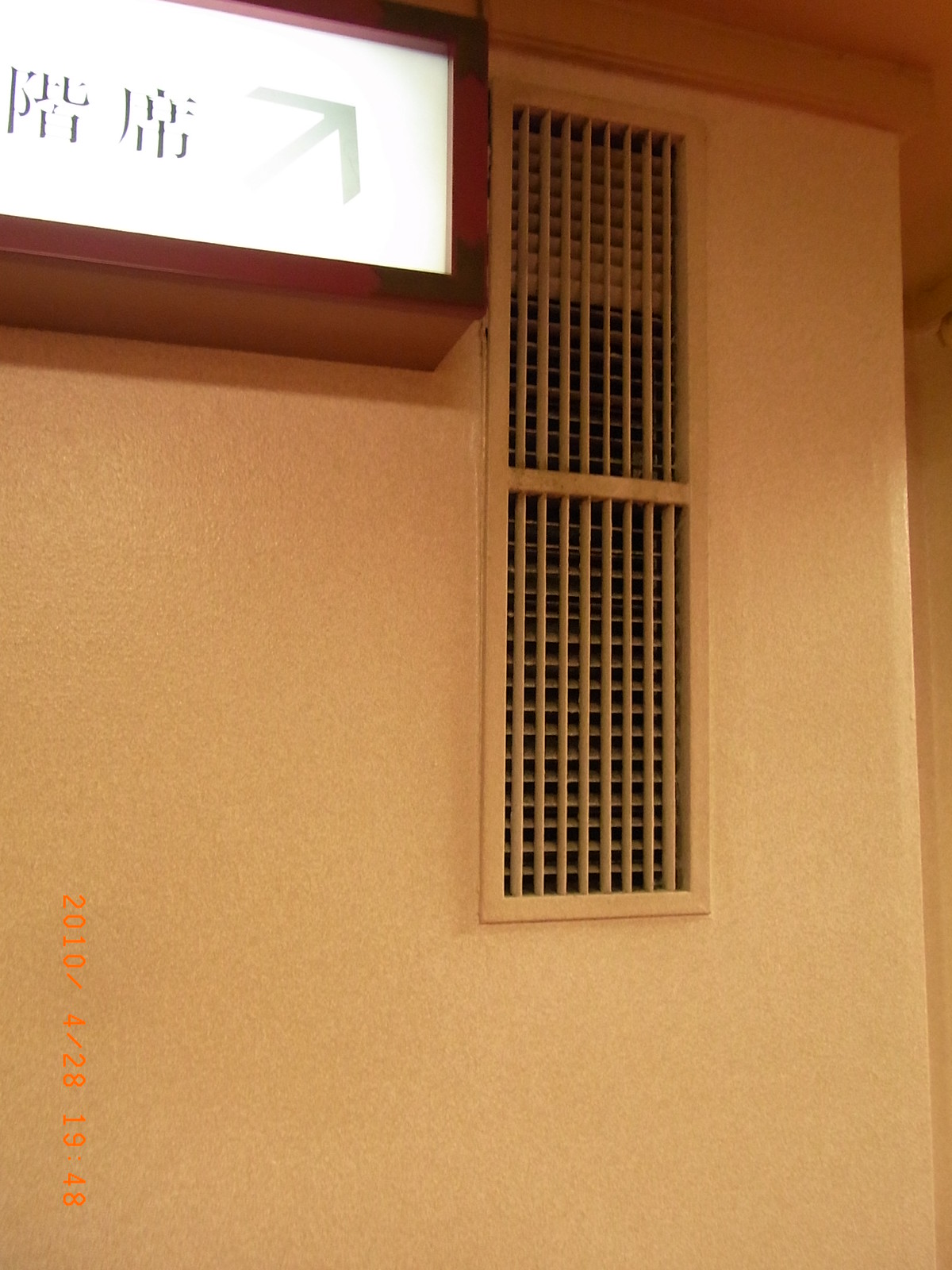The photograph depicts a nondescript, light-colored, potentially beige wall inside a public building, possibly an apartment complex. Dominating the central part of the image is a large rectangular air vent that spans vertically and features a grid of vertical and horizontal slats. Some of these slats appear moveable, with a few tilting upward or downward. In the upper left corner of the image, an illuminated sign is mounted, encased in a darker brown, almost redwood-colored frame. The inner part of the sign is bright white, displaying Asian characters, likely Japanese or Chinese, along with a green-grey arrow pointing diagonally upward to the right. The lower left of the photograph includes an orange-colored date and time stamp reading "2010/4/28 19:48," indicating the photo was taken on April 28, 2010, at 7:48 PM.